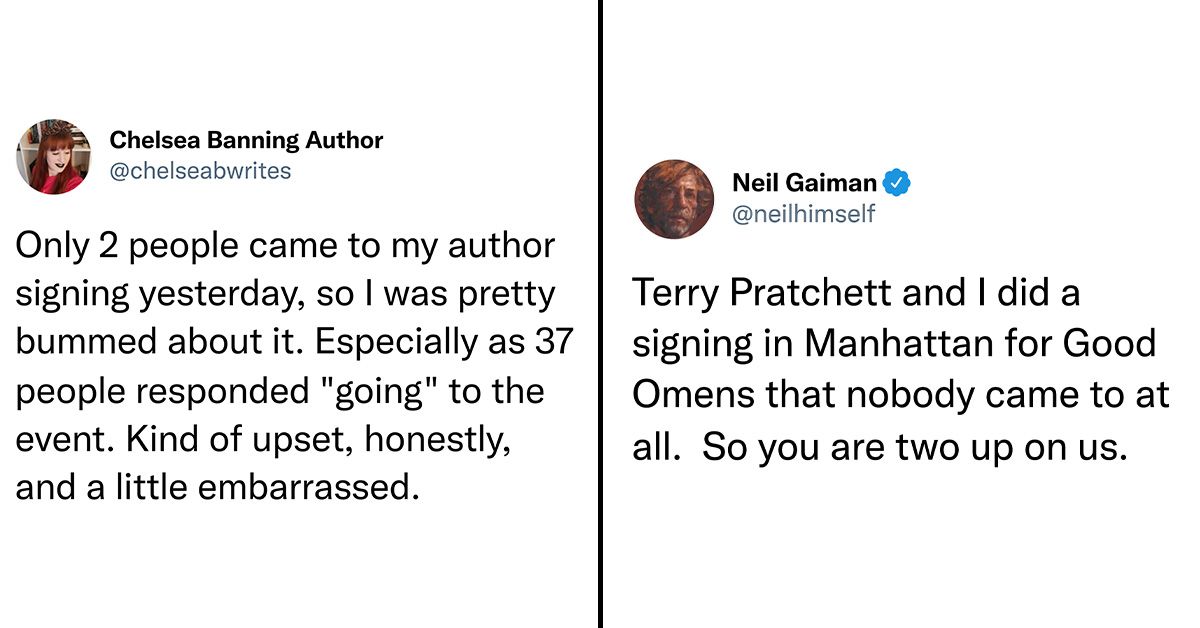The image displays two Twitter posts. On the left, Chelsea Banning Author expresses her disappointment that only two people attended her book signing, despite 37 people RSVPing, leaving her feeling upset and embarrassed. On the right, a verified tweet from renowned author Neil Gaiman responds to Chelsea’s post, sharing a personal anecdote to console her. He recounts that during a Manhattan signing for "Good Omens" with Terry Pratchett, no one showed up, humorously noting that she did better than they did by having two attendees. Neil's supportive response highlights both empathy and humility.